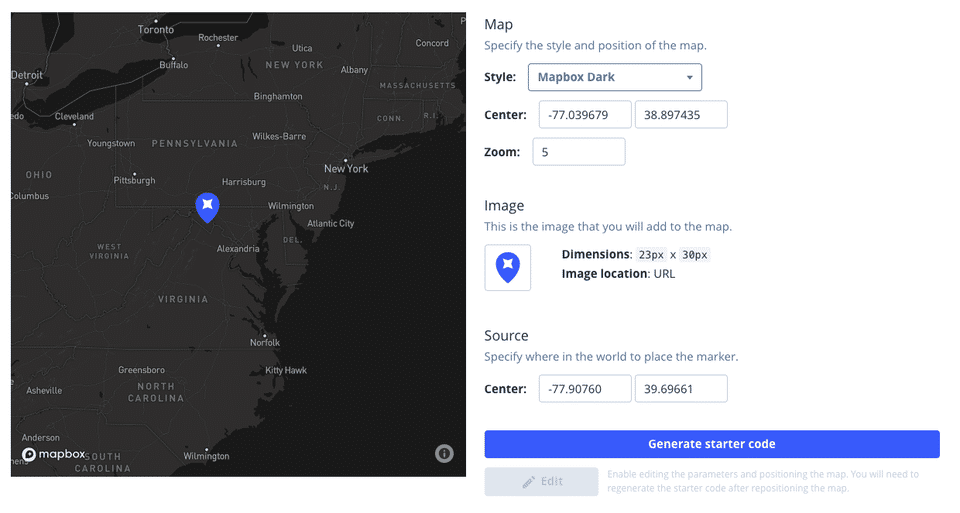A detailed screenshot showcases a map interface with various options and settings. The map itself is prominently displayed on the left side, encompassing regions such as Pennsylvania, Virginia, North Carolina, New York, Connecticut, and Massachusetts. On the right side, a set of controls is visible at the top, beginning with a label "Map" alongside instructions to "specify the style and position of the map." The specified settings include "Style: Mapbox Dark," a centered map view, and geographical coordinates indicating the area's central point. Additionally, the zoom level is set to 5. Below these settings, another section labeled "Image" is present, outlining details about the image to be added to the map, including its dimensions and location. The source input prompts for the marker's specific placement on the map, indicating where exactly in the world the marker should be positioned.